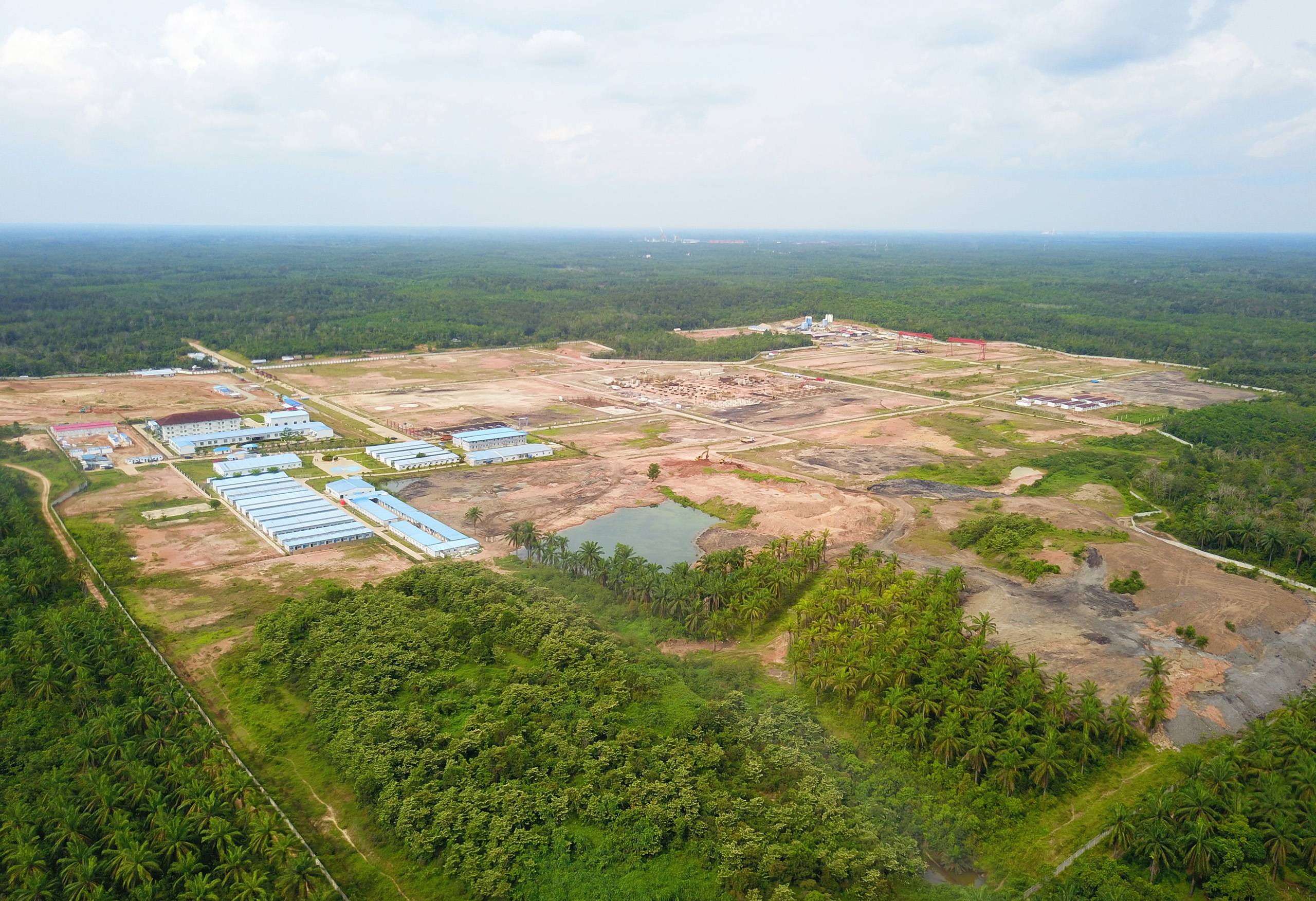This aerial photograph captures a construction site set amidst a verdant expanse of palm trees and forests. The site features a stark contrast between the lush greenery and the expansive brown, flat dirt area. Distinct roadways crisscross through the excavation site. On the left side, a cluster of completed structures, likely garages and apartment buildings, are visible along with a series of long, uniform buildings. On the right side, new buildings are under construction. Dominating the center of the site is a water-filled quarry or lake, its small, square shape standing out against the brown landscape. The sky above is light gray with white clouds, further highlighting the stark contrast between the green surroundings and the cleared, brown earth of the construction area.